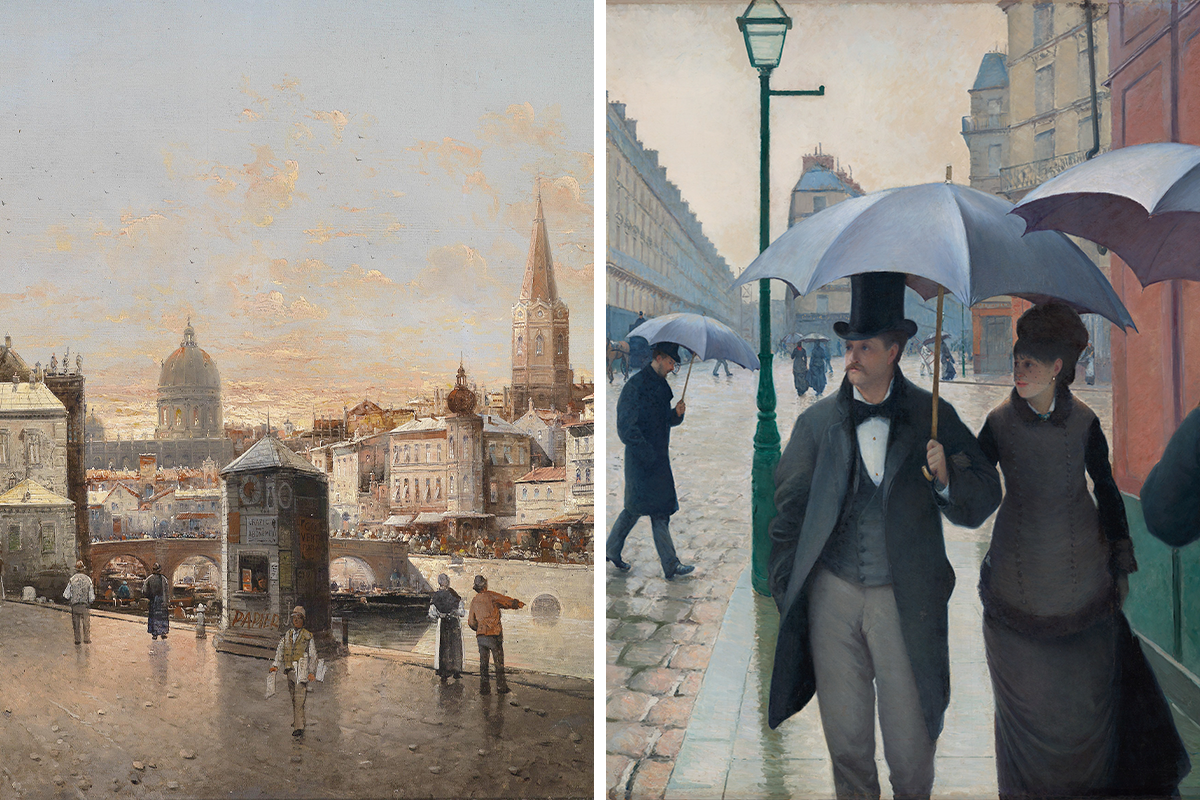In this image, we see two distinct paintings displayed side-by-side, each capturing different urban scenes. The painting on the left depicts a sepia-toned cityscape, likely Paris, featuring a busy river canal crossed by a bridge adorned with several black boats. In the foreground, a young man attempts to sell newspapers near a booth marked with the red-lettered word "Papier." The pathway beside the river is dotted with several people moving about. The background showcases an array of buildings, including a prominent church steeple and a domed structure rising high against the skyline.

On the right, the scene shifts to a more vividly colored urban setting. This painting, leaning towards a realistic style, illustrates a man in a sophisticated black tuxedo and top hat, holding an umbrella with a blue top in his left hand. Beside him is a woman in a black dress, grasping his arm as they stroll down a street. They are surrounded by a handful of other pedestrians, also carrying umbrellas, as they navigate the city square. The sky is depicted in a striking yellow hue, and behind them, vibrant red, green, and blue buildings add a lively backdrop to the scene. A green street lamp further accentuates the urban ambiance.